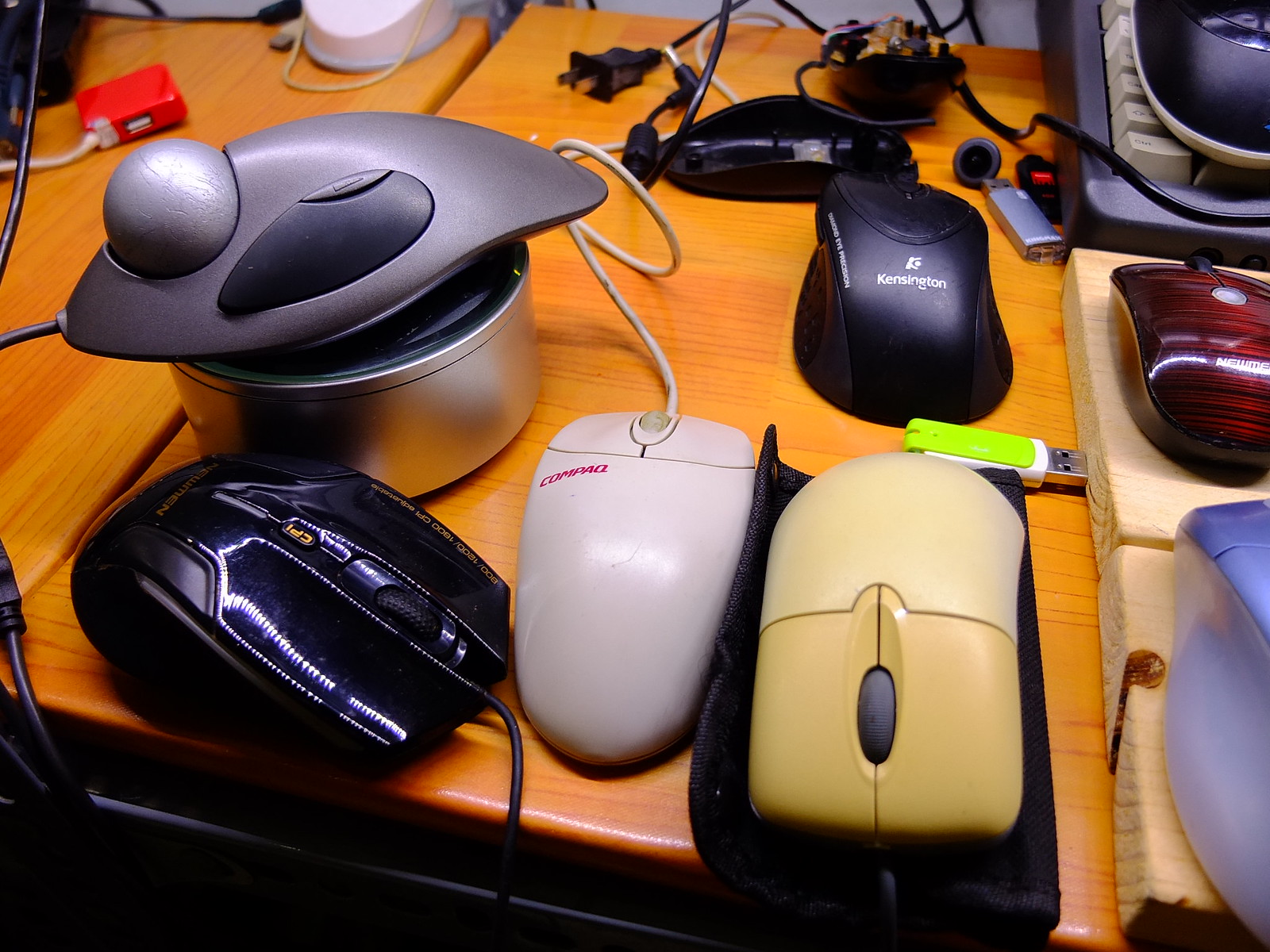The photograph showcases a cluttered wooden tabletop, crafted from reddish maple wood, covered with an array of outdated computer mice. In the upper right corner, a purplish-colored keyboard is partially visible. The table displays a mix of eight distinct mice, including a marbled red one, a dingy tan one, a black gaming mouse with a shiny, possibly leather finish, and an old model with a top-mounted trackball. There are also several black mice, a white one labeled "COMPAQ" in the middle, and a few colorful ones such as light blue and pink. A silver mouse sits atop a tin. Strung cables and cords further add to the chaotic arrangement, reflecting a collection of vintage devices from the early 2000s.